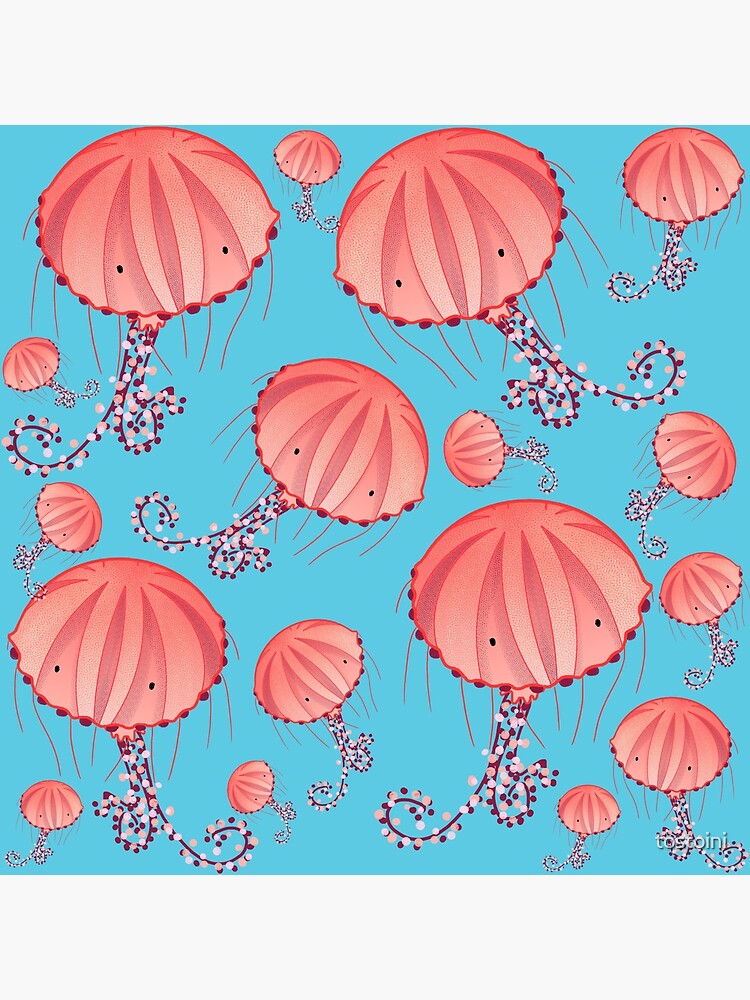This image features a whimsical, idealized depiction of cartoonish jellyfish set against an aqua or light blue background, giving the impression of an underwater scene. Each jellyfish has a pink to reddish dome with two black eyes, adding a touch of character to their appearance. Their tentacles, extending below, are adorned with colorful beads in shades of pink, blue, and brown, suggesting movement and a playful nature. The jellyfish vary in size, with some appearing closer and larger, while others are smaller, creating depth within the image. In the bottom right corner of this charming illustration, the name "Tostoini" is inscribed, adding a signature touch to the artwork.